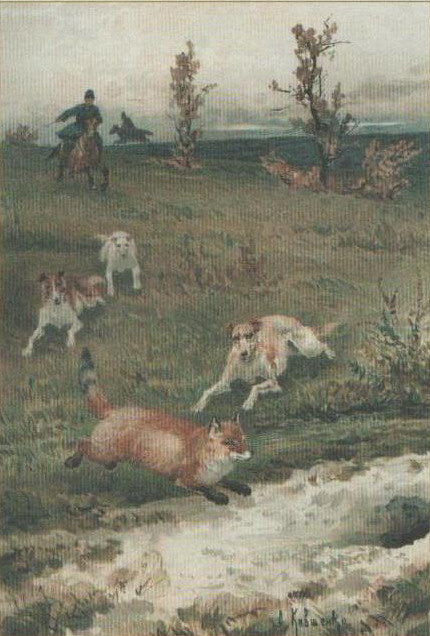The painting, rendered in an 18th-century European style with muted, weathered colors, showcases a classic fox hunt. Centered in a vertical, rectangular frame, it captures a vibrant scene of a red fox darting across a lush, green field, its dark brown paws and white neck contrasting against the greenery. Chasing the fox are three distinct hunting dogs: one solid white, another dappled brown and white, and a mostly white dog with touches of brown. 

In the background, atop horses, are a few riders—including a soldier, possibly Napoleon, identifiable by his helmet and whip—trailing the dogs. The terrain is hilly and adorned with scattered trees and bushes, exuding an old-world charm. A cloudy, white sky looms above, adding to the scene's dramatic tension. In the distance, hints of serene water and faint mountains complete the picturesque landscape. Notably, the bottom right corner reveals a foxhole, suggestive of the fox's desperate escape route, enhancing the painting’s dynamic narrative.